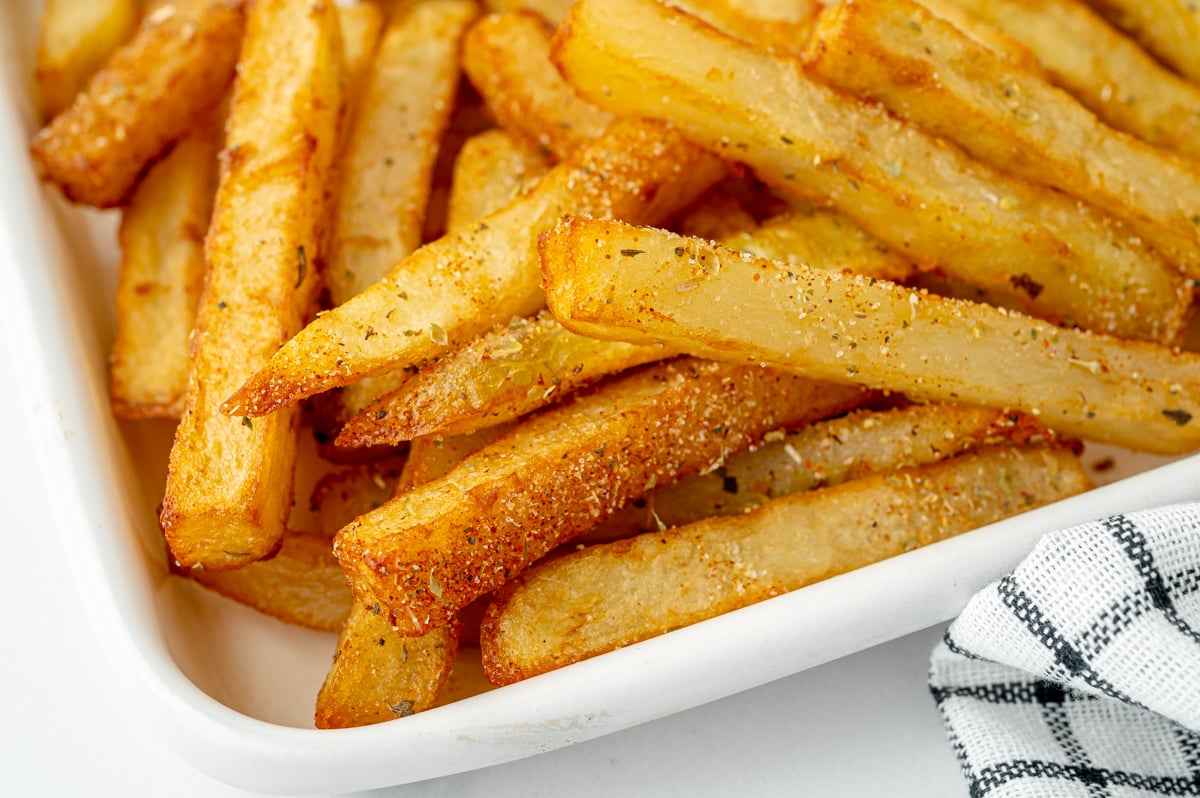This close-up photograph captures a mouthwatering array of golden French fries, perfectly seasoned with a mix of salt, reddish-orange spices, and dark green herbs, hinting at Italian flavors. The fries lie invitingly in a white rectangular dish, their soft yellow and golden hues gleaming with a slight sheen of oil, testament to their crispy texture and the browning on the edges. The bottom right-hand corner of the image features a green grid-patterned and white plaid dishcloth, adding a touch of domestic charm to the scene. Set against a pristine white table, this brightly lit image emphasizes the freshly prepared appearance of the delectable fries, making it ideal for an advertisement, food magazine, or restaurant display.